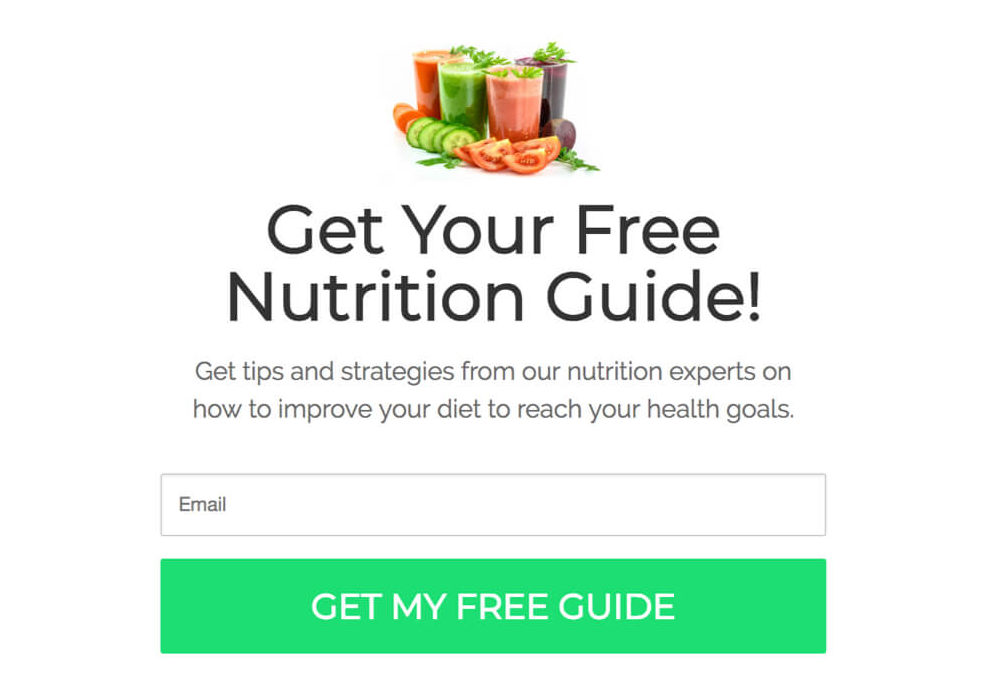This screenshot showcases a sign-up page for an email subscription service with a clean, white background. Dominating the center of the page is a vibrant logo featuring four tall glasses filled with different fruit juices. The tomato juice is prominently displayed in the front, flanked by cucumber juice on the left and beet juice on the right, with strawberry juice positioned slightly behind the cucumber juice on the left side. Below the graphic, bold black text declares, "Get Your Free Nutrition Guide," accompanied by a subtext in a smaller font that reads, "Get tips and strategies from our nutrition experts on how to improve your diet to reach your health goals." At the bottom of the page, there is a small input bar for the email address and a blue-green button labeled "Get My Free Guide." Overall, the page maintains a minimalist design with a focus on the colorful juice graphic and the essential call-to-action elements.